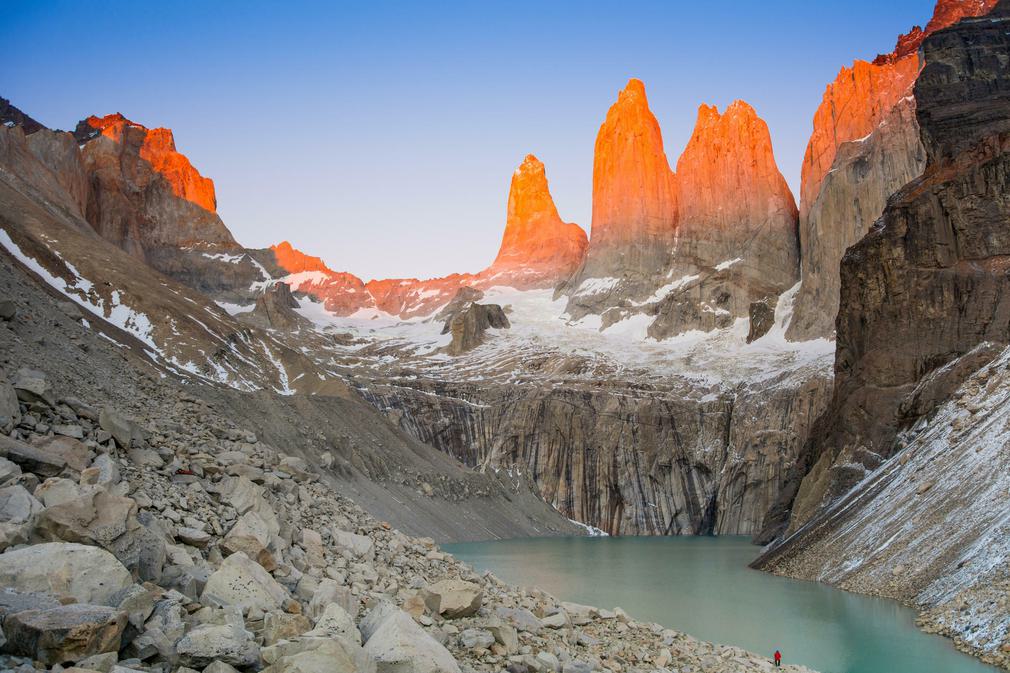The photograph depicts a large desert canyon with a striking juxtaposition of white sandy walls and rugged brown rock formations. Central to the image is a vibrant greenish body of water, which pools at the base of these dramatic cliffs. In the background and extending high into the sky, the rocks transition into towering, sharp peaks bathed in a brilliant orange hue, likely from the sunlight. Some snow can be seen adorning the lower levels of these peaks, both on the left and right sides of the canyon. At the very top, a cloudless sky fades from a bright blue to a deeper, darker shade. In the lower right corner, a diminutive figure in a red shirt or jacket accentuates the immense scale of the landscape, barely noticeable against the vast rocky mountainside.